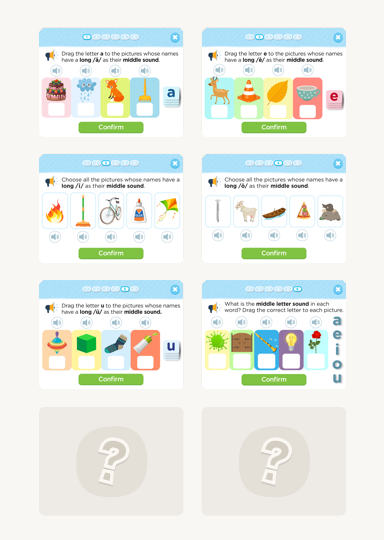Screenshot of an interactive educational activity designed like flashcards with a colorful, child-friendly interface. The layout features two columns and four rows, each populated with various questions and answers to engage primary school children in phonics learning. The top section has three rows showcasing vibrant illustrations accompanied by a speaker icon above each image, allowing users to hear the corresponding sounds. Examples include illustrations of a cake, cloud, rain, fox, and brush. At the top, instructions direct learners to "drag the letter A to the pictures whose names have a long 'a' sound in their middle sound." Students interact by dragging the letter 'A' into designated white boxes under the images. Once selections are made, a green button at the bottom allows them to confirm their answers.